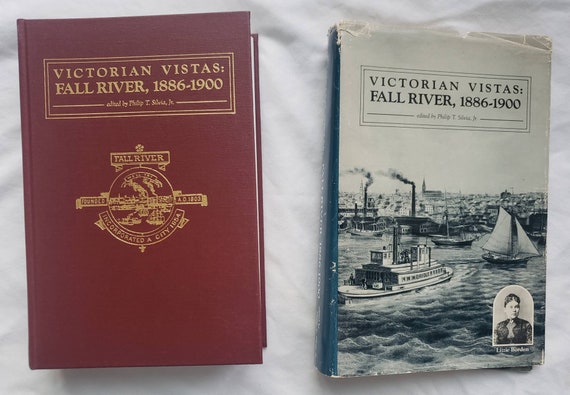The image displays two hardback books on a light gray, slightly rippled fabric background. 

The book on the left has a thick, dark burgundy cover. At the top, it features a rectangular box with a double gold outline. Inside, in capitalized gold letters, it reads "VICTORIAN VISTAS; FALL RIVER, 1886-1900." Beneath this, though difficult to read, is some small text likely indicating the editor. Further down, there is a round gold logo. At the top of the logo, "FALL RIVER" is visible, with additional indistinct banners to the sides. The bottom of the logo reads "INCORPORATED A CITY 1854."

The book on the right has a worn cover jacket, with its left side in blue and the rest in gray. The top features the title "VICTORIAN VISTAS, FALL RIVER, 1886-1900" in black letters. The cover shows a picture of a steam engine traveling down a river with boats. Additionally, there is an image of a woman in the lower right corner.